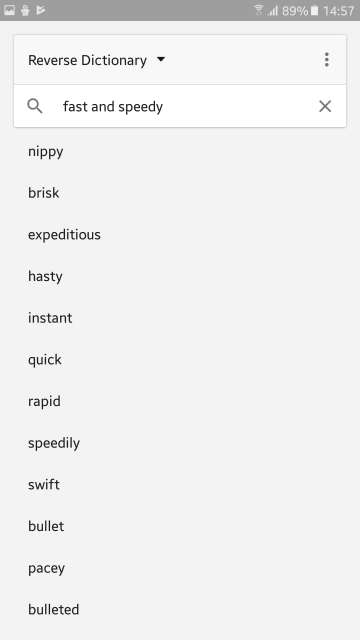This is a detailed screenshot from a smartphone interface. The top half-inch of the screen features a dark gray status bar. Below this, the background transitions to a light grayish-blue color. On the top left of the status bar, there are three icons: a picture icon, a person icon, and the Play Store icon. Moving to the right, the status bar displays the time "14:57," a white battery icon showing 89% charge, and full signal Wi-Fi and internet icons.

Just below the status bar, there is a light blue rectangular section with the text "Reverse Dictionary," accompanied by a small black downward-pointing triangle. Three vertical dots are aligned next to this section on the right side, indicating a menu option.

Further down, there is a white rectangular search bar featuring a search icon on the left and the phrase "fast and speedy" inside it. An "X" icon is located on the right side of the search bar, likely for clearing the text.

Beneath the search bar, the background changes back to light blue and presents a list of words related to the search term. The words are:

1. Nippy
2. Brisk
3. Expeditious
4. Hasty
5. Instant
6. Quick
7. Rapid
8. Speedily
9. Swift
10. Bullet
11. Pacey
12. Bulleted

These words are displayed in lowercase black lettering. This light blue section with the words occupies roughly an inch of screen space horizontally, while the remaining portion of the screen returns to the solid light grayish-blue color.